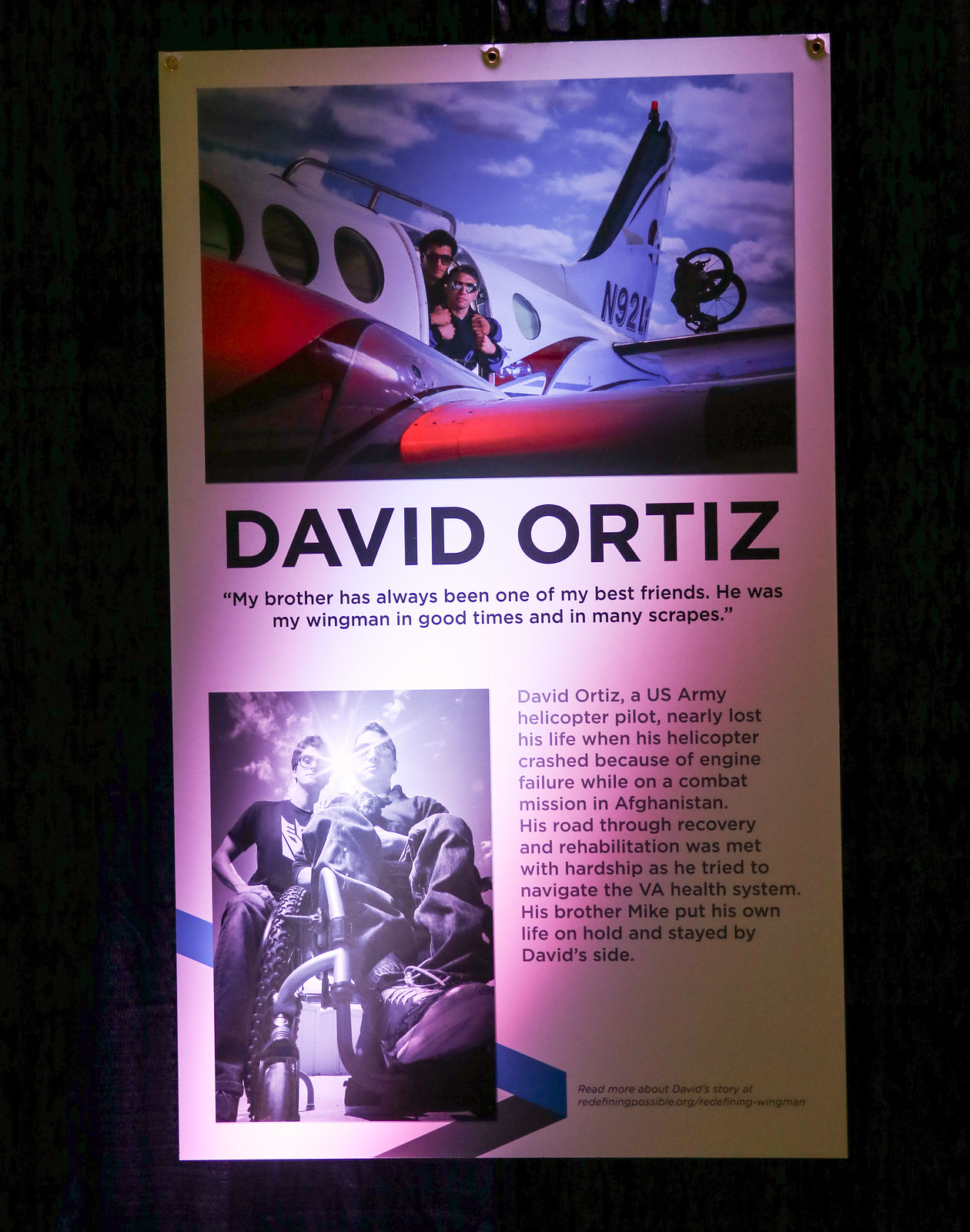The poster, illuminated with white and purple lighting, presents a heartfelt tribute to U.S. Army helicopter pilot David Ortiz, who nearly lost his life due to an engine failure during a combat mission in Afghanistan. The top section features a poignant quote, "My brother has always been one of my best friends. He was my wingman in good times and in many scrapes," beneath which the name David Ortiz appears prominently. Flanking this quote is an image of two young men, presumably David and his brother Mike, peeking out of the doorway of a small airplane under a clear blue sky. Below this, another black and white photograph depicts David in a wheelchair, accompanied by Mike, who dedicated himself to David's recovery and rehabilitation. The narrative outlines the severe challenges David faced within the VA health system post-accident and underscores Mike's unwavering support, emphasizing the profound bond between the brothers. The information concludes by directing readers to learn more about their journey at redefiningpossible.org/redefining/wingman.